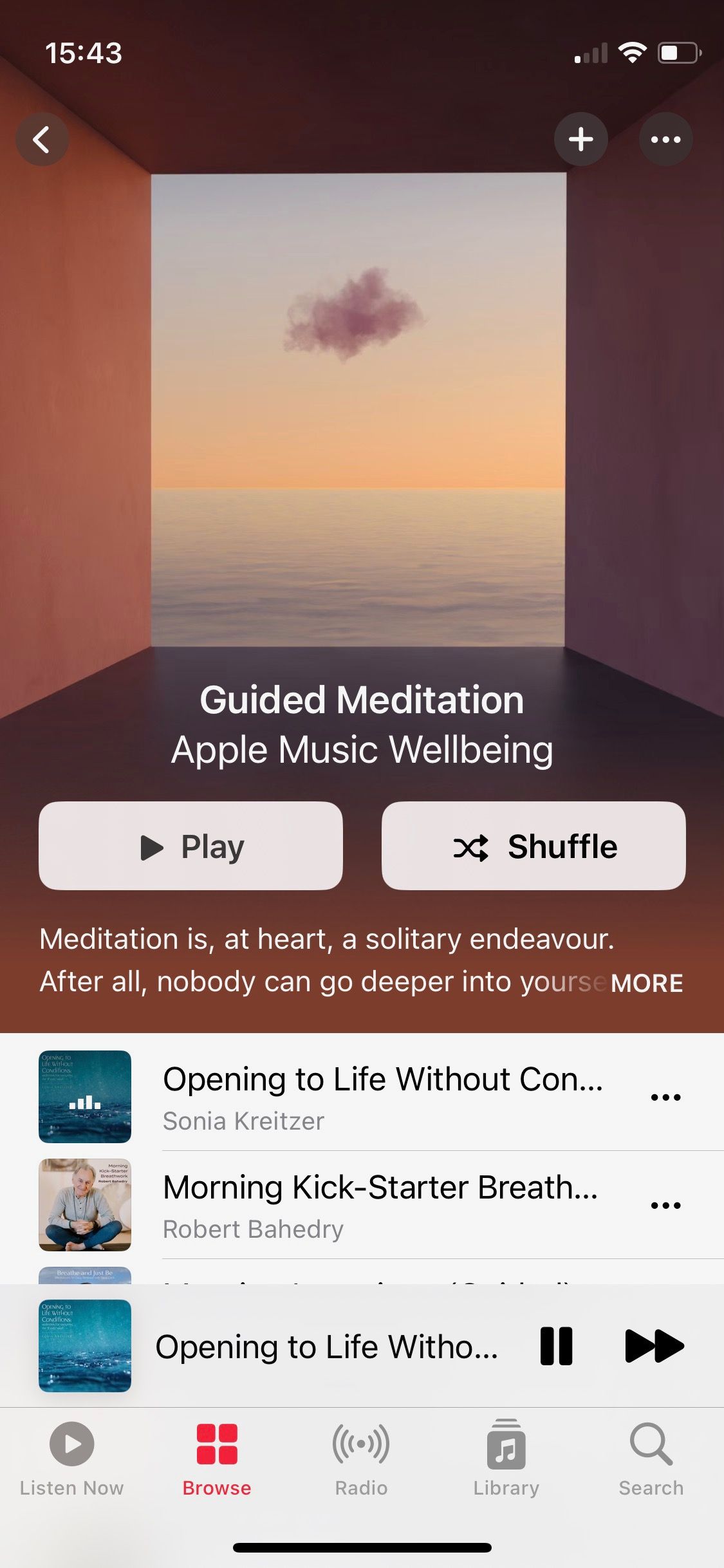This image, taken from a smartphone, displays an app interface with a rectangular orientation, where the longer side spans from top to bottom. At the very top of the screen, the status bar shows the time, "15:43," in white text on the left. To the right, there is a signal strength icon with one bar, a full Wi-Fi signal, and a battery icon that is about half full. Below the status bar are navigation and menu icons, including a left-pointing arrow, a plus sign, and three horizontal dots on the right.

The active app window occupies most of the screen, revealing an ambient scene of a room that opens up to a breathtaking ocean view with a clear sky punctuated by a single cloud. The room has a distinctive copper hue. Below this picturesque view, white text reads "Guided Meditation, Apple Music Wellbeing," indicating the current feature of the app.

Further down, two large white buttons labeled "Play" and "Shuffle" in black text are prominently displayed. Below these buttons, a motivational phrase is featured in white text: "Meditation is at heart a solitary endeavor. After all, nobody can go deeper into yours," with an option to read more presumably available. 

At the bottom of the screen, a greyish box lists various meditation sessions available: "Opening to Life Without Calm," "Morning Kickstarter Breath," and "Opening to Life Without"—the latter cut off mid-title and unviewable in full. The current session being played is highlighted.

Lastly, a menu bar at the very bottom of the screen contains five navigation options: "Listen Now," "Browse," "Radio," "Library," and "Search," facilitating easy navigation through the app.